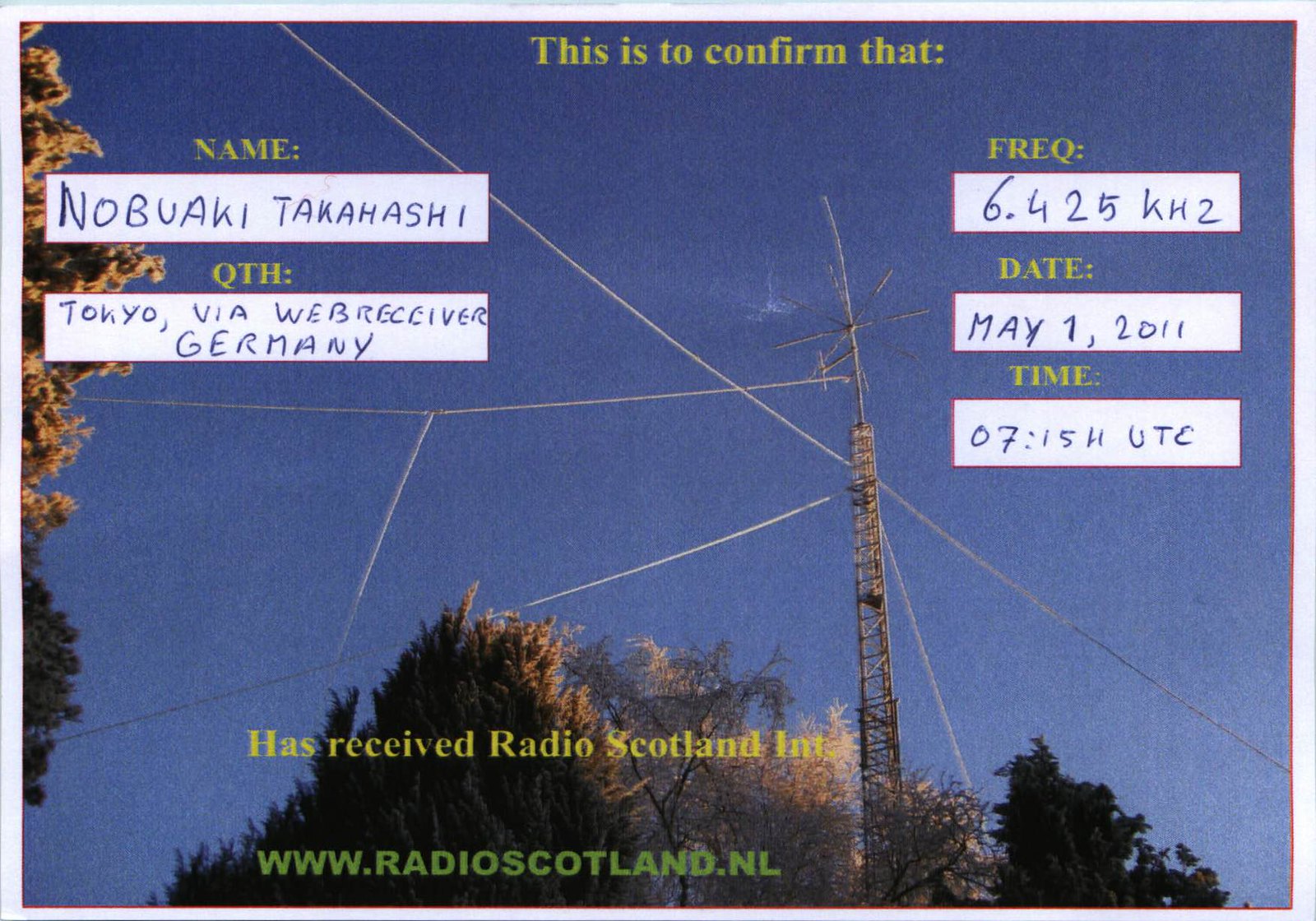This detailed image, which appears to be a printed postcard or photograph, captures a view looking up towards a large radio tower positioned centrally against a blue sky. The skyline dominates the image, while trees frame the scene from the left side and bottom. The radio tower features long support ropes extending towards the ground, with power lines also visible crossing the scene. 

The top portion of the image contains yellow text reading, "This is to confirm that," followed by handwritten entries for "Name: Nobuaki Takahashi" and "QTH: Tokyo via Web Receiver Germany." On the right side, fields for "Frequency," "Date," and "Time" are filled in with "6.425 kHz," "May 1, 2011," and "0715 UTC," respectively.

In green capital letters at the bottom of the image, overlaying the trees, it states, "Has received Radio Scotland International," followed by the website "www.radioscotland.nl." The overall setting appears to be outdoors in the middle of the day, emphasizing an international radio signal confirmation received by Nobuaki Takahashi.